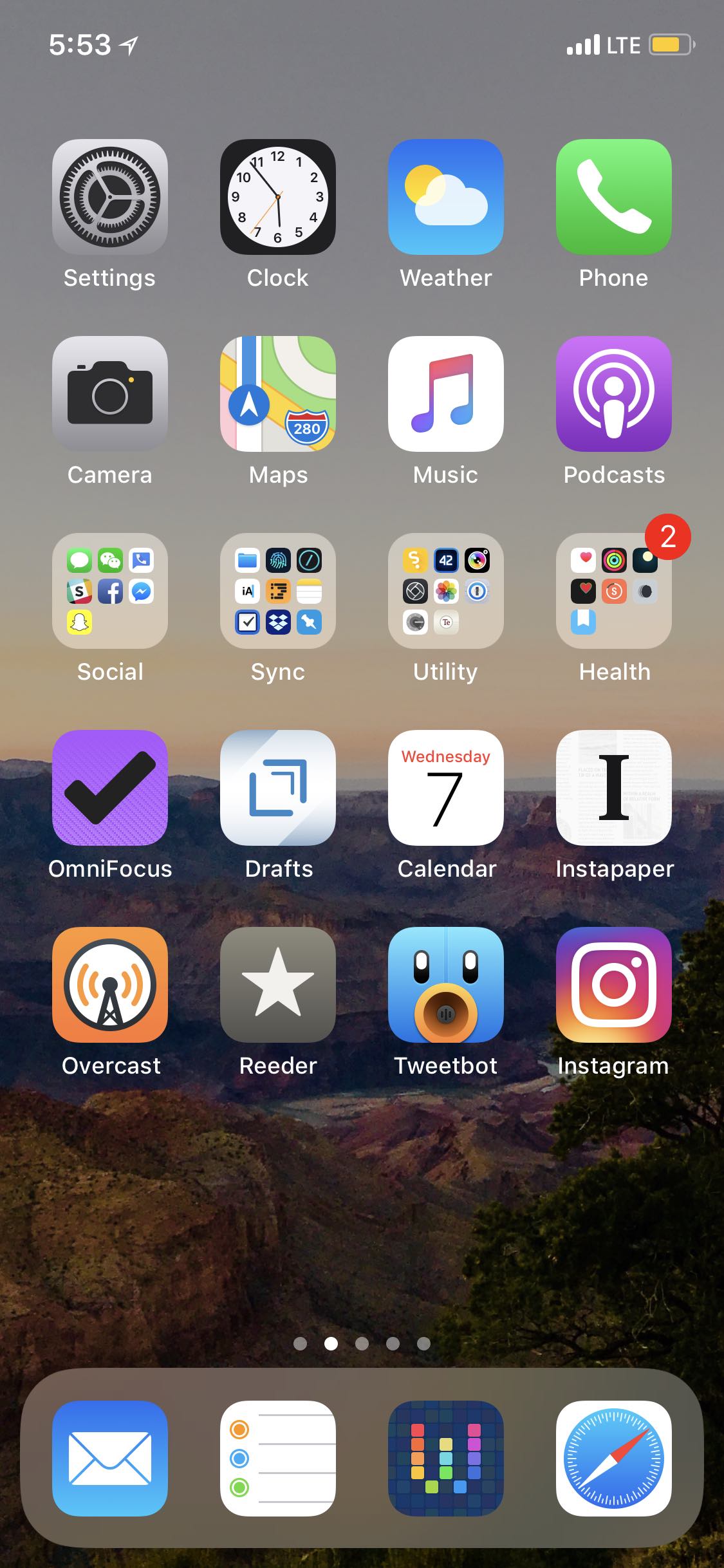This image is a screenshot of a smartphone home screen taken at 5:53 AM. The battery indicator shows approximately 80%, and the signal strength shows four bars. The background image appears to be a stunning landscape of the Grand Canyon during either sunrise or sunset, filling the screen with warm hues and dramatic shadows. There are five rows of four app icons each, neatly arranged in a grid.

- **Row 1**: Settings, Clock, Weather, Phone
- **Row 2**: Camera, Maps, Music, Podcast
- **Row 3**: Social, Sync, Library, Health
- **Row 4**: OmniFocus, Drafts, Calendar, Paper
- **Row 5**: Overcast, Reader, Tweetbot, Instagram

At the bottom of the screen, there is a gray dock which contains three main icons: a blue square with an envelope (likely for email), and an icon depicting a compass. Each app on the screen is represented by a square icon with distinct graphics, making for a visually organized and user-friendly interface.